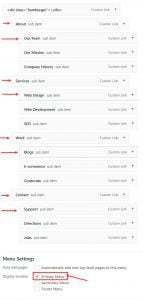The image is an extremely blurry screenshot from a cell phone, characterized by its long and vertical format. The overall background of the image is white, and all the text appears in black, though it is illegible due to the high level of blur and small font size. The most noticeable colored elements are red arrows pointing to specific words within the text.

At the top of the screenshot, there seems to be some sort of heading or title, and to its right, there's an icon resembling a menu toggle button. Each line of text within the column has a small plus sign next to it, perhaps indicating tags or menu options, though these are also not readable. 

The bottom part of the screenshot displays the words "menu settings" clearly, as they are slightly larger in size compared to the rest. Directly above this, a section of text is highlighted with a red rectangular outline, though the contents remain indistinct. Overall, the image appears to depict a menu or list of items, but the excessive blur makes it impossible to decipher any specific details.